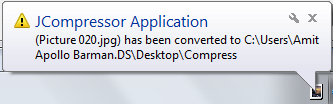The image is a small, rectangular notification screenshot, approximately half an inch to three-quarters of an inch tall and about three inches wide. It features a grey background and appears to originate from the Windows 7 operating system. At the top of the notification, there's a yellow triangular warning symbol containing a black exclamation point, alongside which reads "JCompressor Application" in a blue, sans-serif font. Below this, the notification text states, "picture 020.jpg has been converted to C:\Users\AmitApolloBarman.DS\Desktop\compress." On the far right of the notification are two icons: a wrench and an X button. A glass-pane taskbar is visible at the bottom of the image, further indicating its Windows 7 origin.